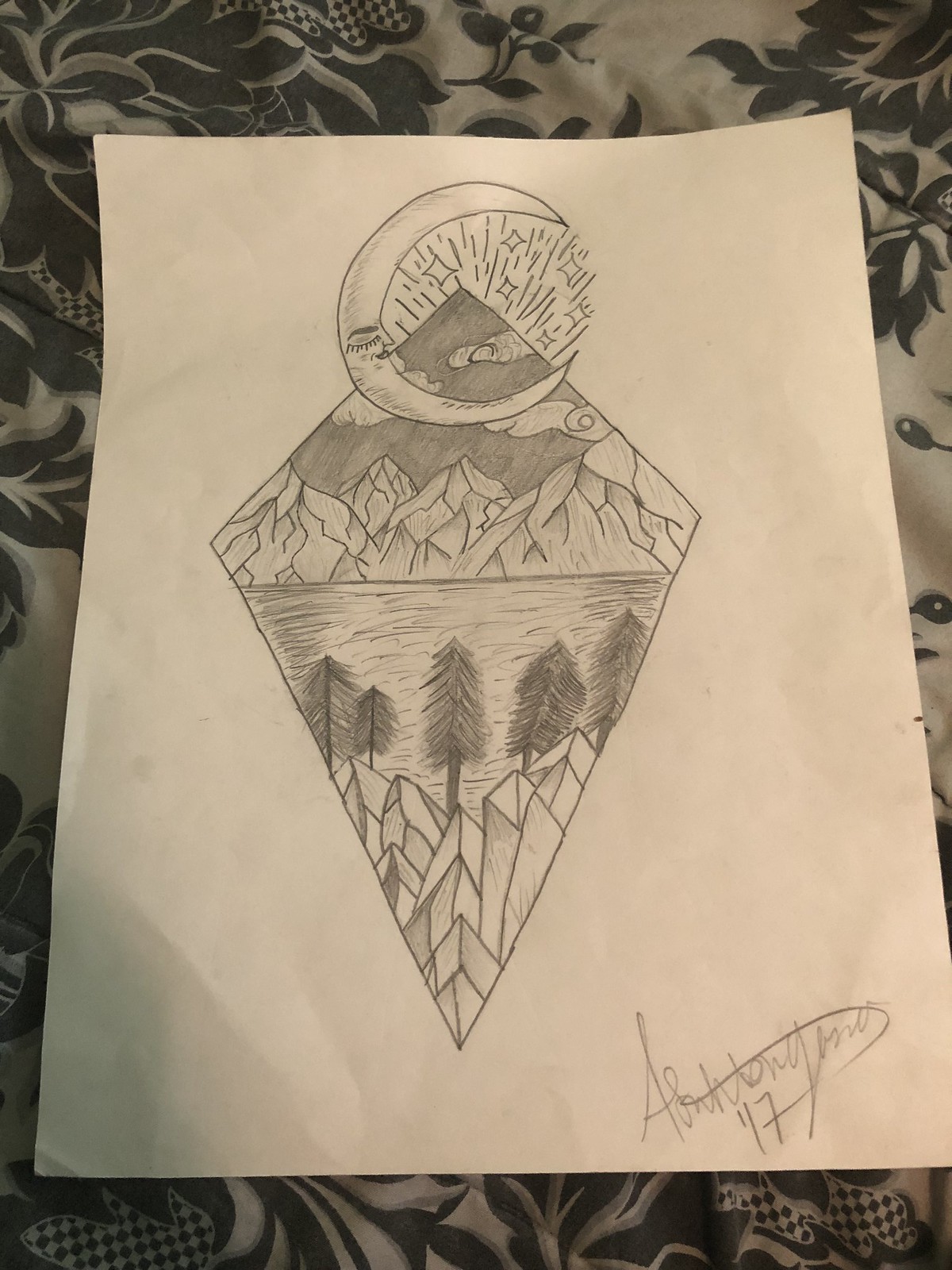This detailed pencil drawing, created on a slightly wrinkled and potentially dirty piece of white paper, features a vertically oriented diamond or kite-shaped composition. The top of the diamond showcases a serene scene with a prominent crescent moon that has feminine features, including eyelashes and a tranquil smile, surrounded by smaller stars and radiant lines that extend upwards, creating a cosmic ambiance. Just below the moon, the diamond's interior top is adorned with intricate and craggy mountainous formations, possibly representing snow-capped peaks or icebergs, with a detailed depiction of clouds shaded darkly in the backdrop.

In the lower portion of the diamond, the landscape transitions to a natural tableau featuring a tranquil lake or river, bordered by large, forested pine trees. Additionally, the foreground includes more craggy, crystal-like features, enhancing the mystique of the scenery. The drawing is completed with the artist’s signature positioned at the bottom right corner of the paper, noting a date that appears to be either 2017 or 1917. The entire artwork is placed on a floral-patterned cloth, adding a subtle touch of delicacy to the overall presentation.